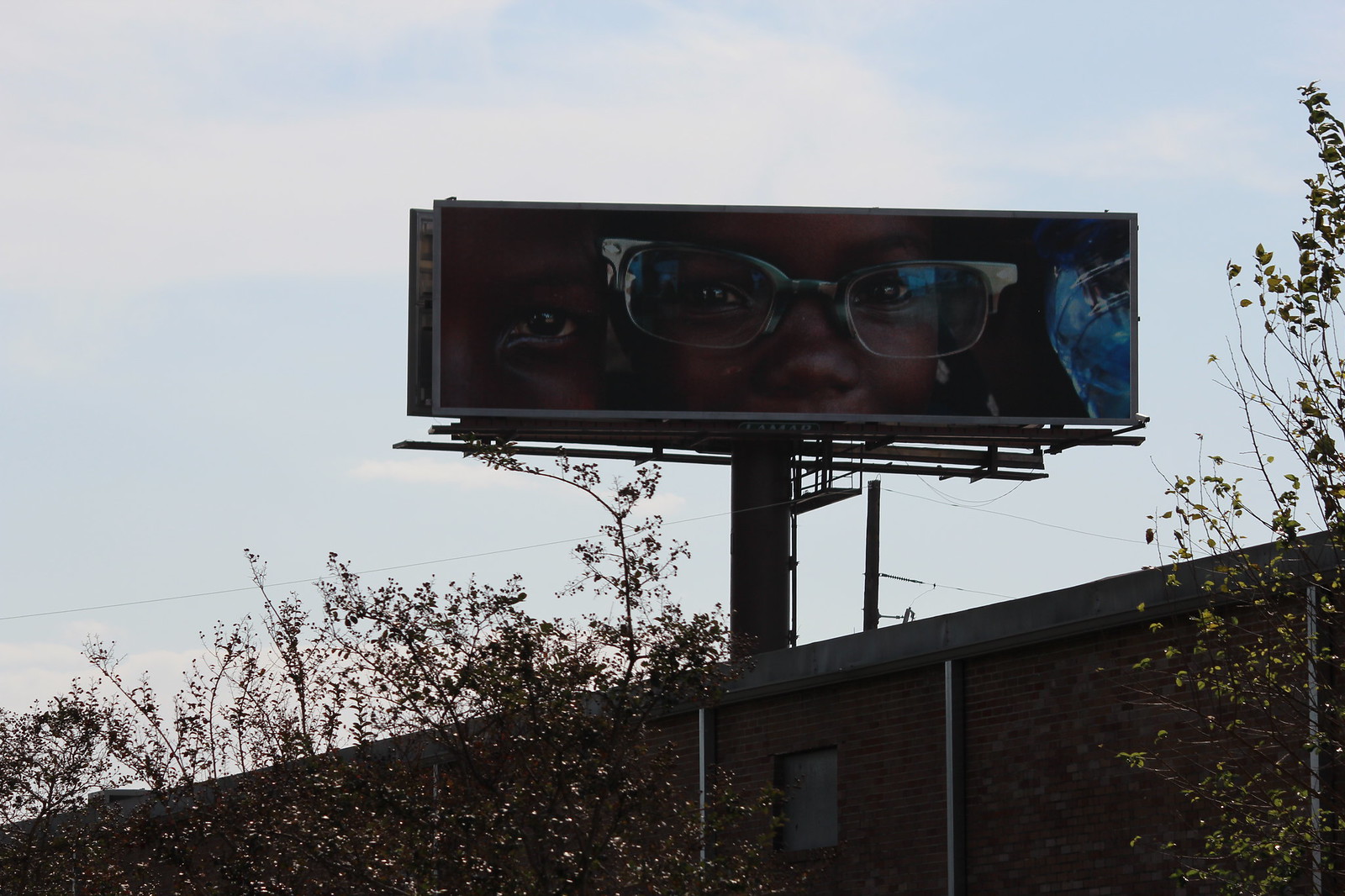The image depicts a close-up of a billboard featuring a young black girl with large, adult-sized glasses. Her head rests affectionately against an adult, of whom only one eye and part of the nose are visible. To the right of the girl, there is a blue object that is unclear. The billboard is mounted atop a red brick building, held up by a short pole. Another billboard is positioned behind it, though its image is not visible. A set of wires runs from a different pole nearby. The building is accented with a line of gray cement at the roof, which is black. A single window is visible on the building, and a backdrop of trees adds a touch of nature to the urban scene.